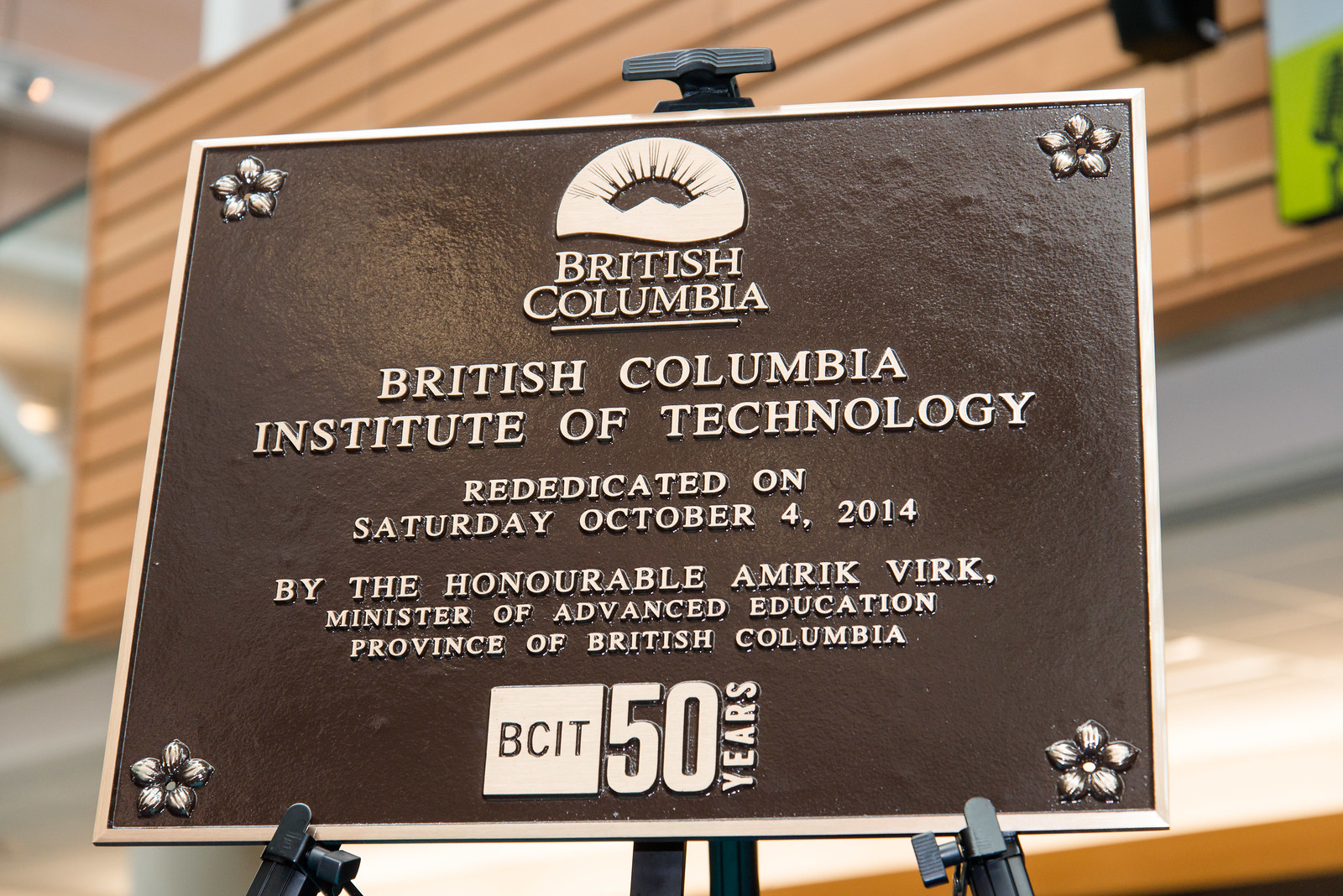The image is a detailed photograph taken indoors, possibly in an art area, library, or office, showcasing a brown metal plaque mounted on an easel stand. The plaque commemorates the British Columbia Institute of Technology, featuring an embossed design with daisies in relief at each corner. At the top of the plaque, a white emblem depicting a sunset or sunrise with mountains is prominently displayed, followed by the inscription "BRITISH COLUMBIA" in large, white, all-capital letters. Below, the text reads "BRITISH COLUMBIA INSTITUTE OF TECHNOLOGY" in an equally bold font. The plaque marks the rededication event on Saturday, October 4th, 2014, officiated by the Honorable Amrik Virk, Minister of Advanced Education, Province of British Columbia. The bottom left features a white box with "BCIT" in brown, and to its right, the inscription "50 years" in white, signifying the institution's milestone anniversary. In the surrounding environment, elements of the building such as brown wooden panels, glass railings, and a green display in the upper right corner can be seen in the background.